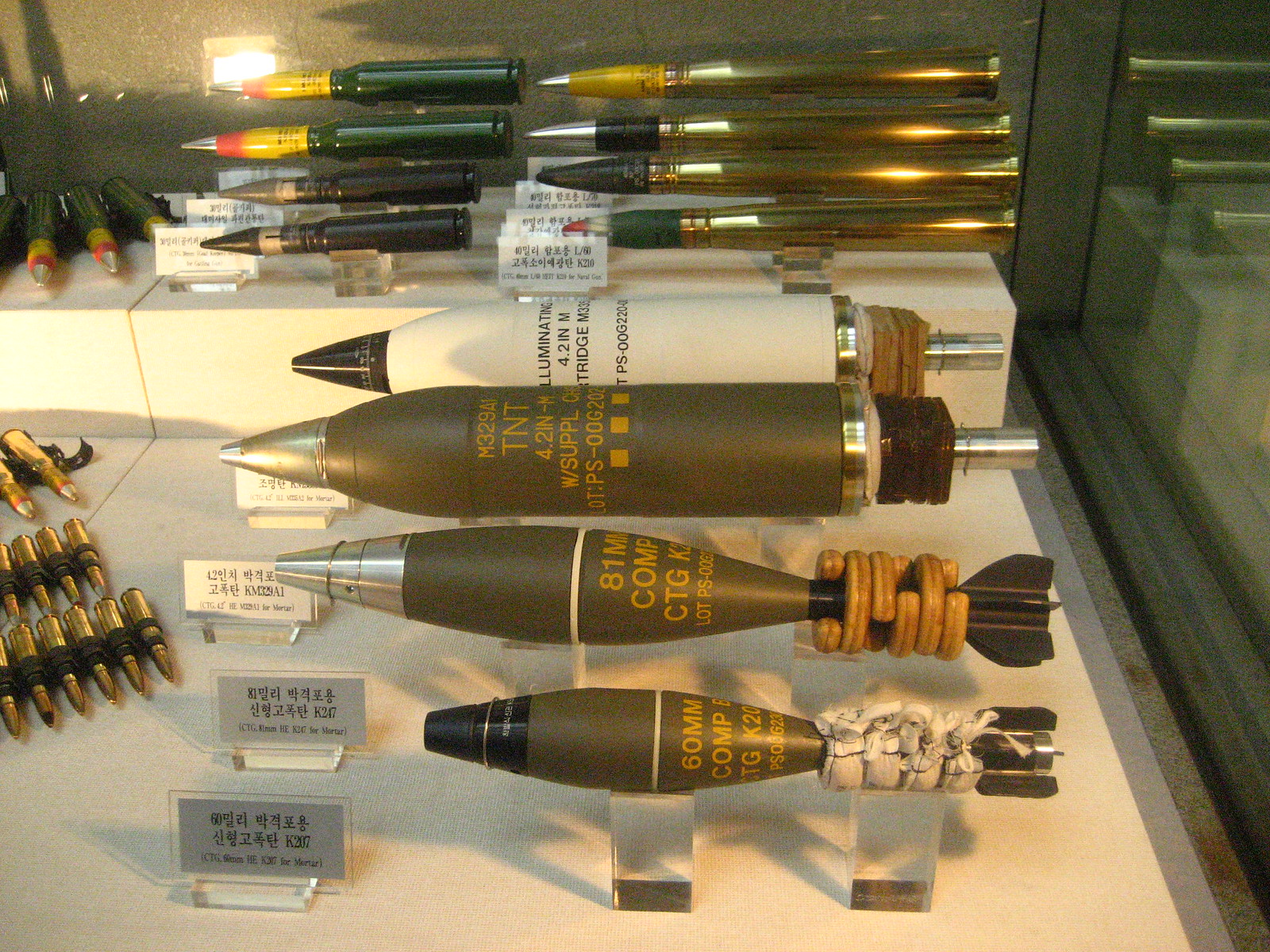The image depicts a section of a museum exhibit, showcasing a collection of military ordnance, likely from a historical period. Central to the display are four vertically stacked objects that resemble bombs or torpedoes. The lowest one is dark green with dark yellow writing and a black tip, while the ones above it are similarly dark green with yellow writing and silver tips. The top-most object is white with a black tip. Behind these, several pointed objects that resemble large bullets are displayed, with varying colors: the rightmost ones are gold with tips in dark green, black, silver, and yellow, respectively. Additionally, adjacent to these are four smaller objects, two in black and two in dark green with yellow tips, and black with a gray tip.

On the left side of the image, there are three organized rows of gold-colored, pointed bullets positioned on a beige platform and encased in glass. Small informational cards are placed in front of each row, likely providing descriptions and historical context. The primary colors observed in the exhibit are gold, green, white, and black. This impressive, well-organized display is housed within a modern museum building, emphasizing both educational and historical significance.